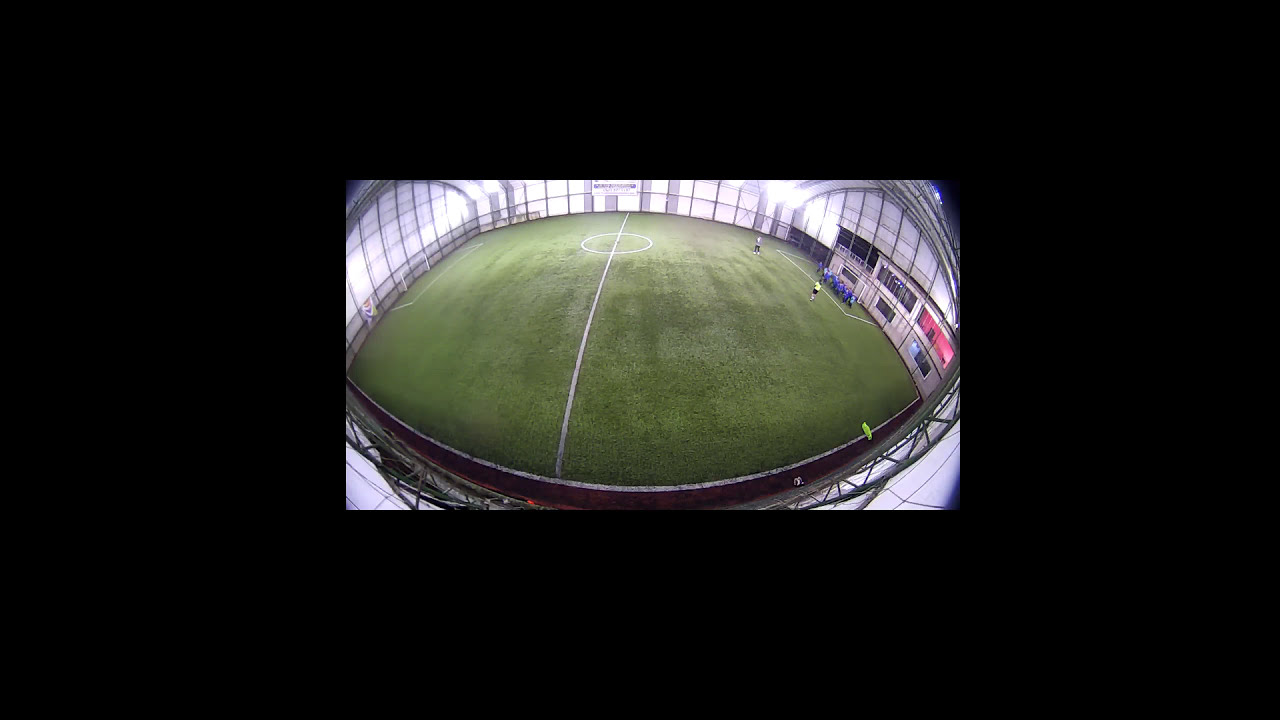The image depicts an indoor soccer facility captured with a fisheye lens, giving it a curvy appearance. The lush, green artificial turf is marked with white lines delineating the boundaries and a perfect white circle at the center of the field. The field is further divided by a midline, and goals are positioned at both ends. Surrounding the field is a structure with many windows and plain white walls framed by black steel girders. On the right side of the field, there is a team in blue uniforms lined up, while a figure in a light lime green jersey with black shorts stands out in the distance. Banners and potentially a scoreboard adorn the walls, alongside a glass dome covering, suggesting a sturdy and illuminated indoor environment. This central soccer field image is set against a larger black rectangular background, enhancing its focus.